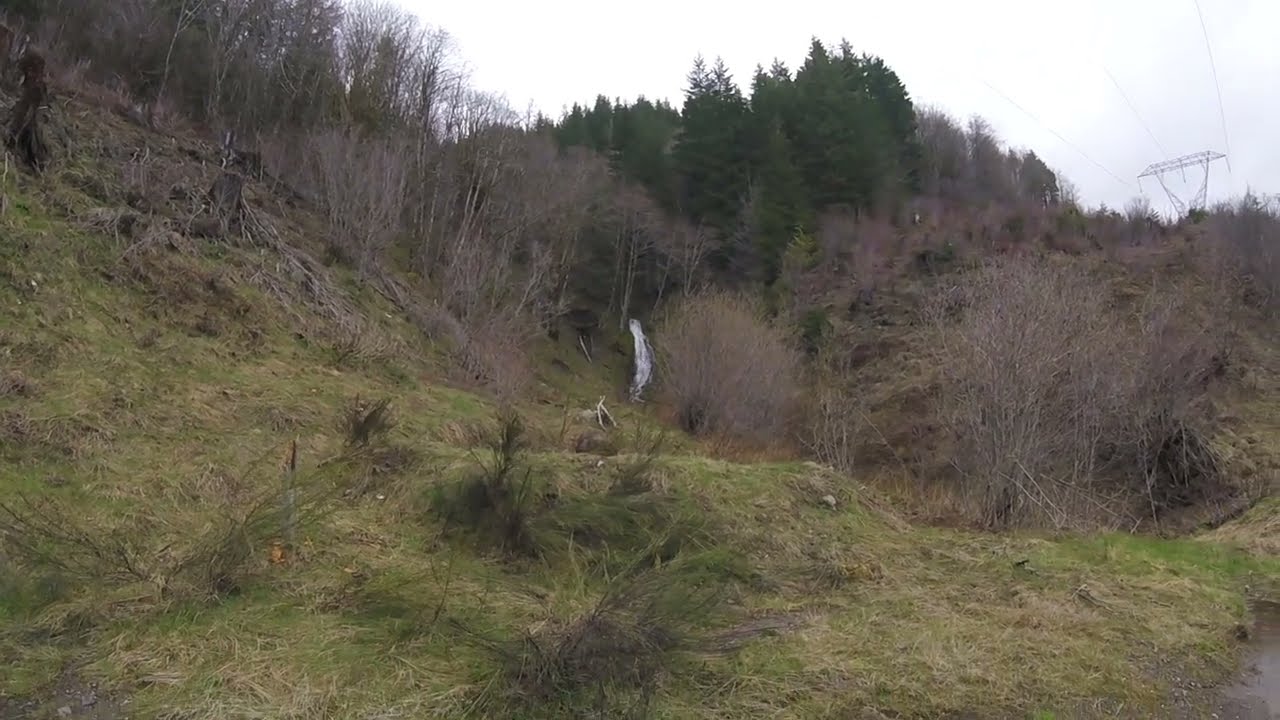The image depicts a desolate hillside, showcasing the transition from late fall to early winter. The foreground is a gentle slope covered in patches of short green grass interspersed with sections of brown, dead grass. In the center of this grassy area, a few clumps of longer green and black ferns stand out, highlighting the uneven terrain with small bumps and plateaus. 

The midsection of the hillside, leading towards the background, features an increasing number of bushes and taller trees. These trees are primarily gray and bare, devoid of leaves. Standing higher in the background, a dense cluster of tall, green pine trees adds a stark contrast to the otherwise bleak landscape. 

On the left side of the image, near the hilltop, more leafless trees stand prominently, their skeletal branches silhouetted against the sky. Meanwhile, the upper right corner of the image reveals black power lines extending from tall metal poles, adding a man-made element to the natural setting.